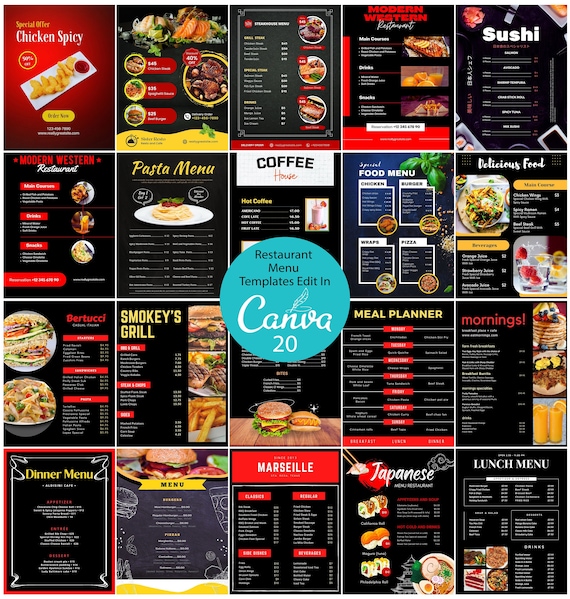This image showcases an advertisement for Canva, presenting a variety of restaurant menu templates that can be edited in Canva 20. The central focal point of the image is a teal circle, prominently displaying the text: "Restaurant Menu Templates. Edit in Canva 20." Surrounding this circle is a 5 by 4 grid, featuring 20 diverse menu templates. 

The menus are predominantly in shades of red and black, with accents in either yellow or red, giving them a vibrant and professional appearance. Each template caters to different types of cuisine, including options for sushi, pasta, coffee, modern Western, Smoky's Grill, Japanese, lunch, and breakfast. For example, there's a bright red "special offer chicken spicy" menu featuring a tempting plate of chicken tenders with sauce, and another for a Japanese restaurant showcasing appealing images of food. Some menus feature just text, such as a meal planner listing items without images, and a sushi menu with minimal graphics apart from a small picture in the upper left corner.

Overall, the array of templates highlights the versatility and range of Canva's design options, suitable for a wide spectrum of dining establishments.